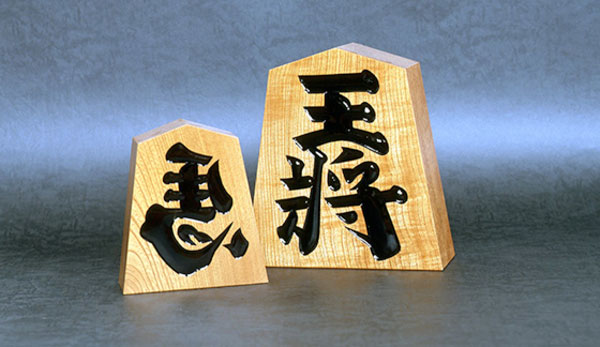The image depicts two angular, light brown wooden blocks, reminiscent of tombstones, positioned against a gradient background that transitions from blue at the top to gray at the bottom. Both blocks exhibit prominent wood grain and bear black-painted Chinese characters. The blocks, differing in size, feature five sides: a point at the top, two angled sides, and a straight base. The larger block is slightly behind and to the right of the smaller one, overlapping at the bottom right corner. The background hints at a metallic, reflective surface, contributing to the contrast with the wooden textures and engraved characters.